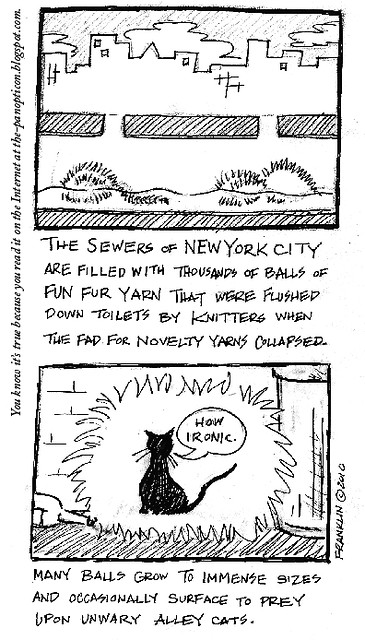This black and white cartoon strip features two panels with text between and around them. The top panel illustrates a cityscape with buildings, a wall, and some bushes in the foreground. Beneath this image, the caption reads: "The sewers of New York City are filled with thousands of balls of fun fur yarn that were flushed down toilets by knitters when the fad for novelty yarn collapsed." A diagonal text from the bottom panel up to the top reads, "You know it's true because you read it on the internet at the Panopticon blog." The bottom panel depicts a black cat sitting near a trash can with bushes around it. A speech bubble above the cat says, "How ironic," while a spiky circle around the cat highlights its comment. The final caption below this scene adds, "Many balls grow to immense sizes and occasionally surface to prey upon unwary alley cats." This detailed and eccentric comic mixes humor with an imagined urban legend.